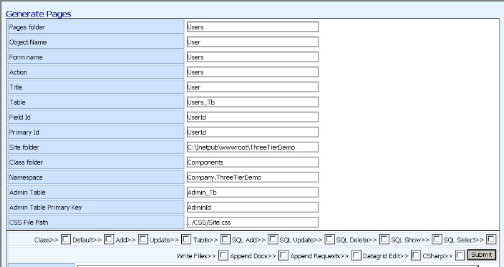The image is a blurred screenshot from an outdated web page, presumably used by IT professionals. The design and font styles suggest that the page is at least a decade old, originating from the early to mid-2010s or perhaps even earlier. The interface features a predominantly white background, with a section on the left occupying roughly one-third of the screen. This section is highlighted in a very light sky blue color. The top border is an even lighter shade of blue, almost greenish.

On the left side, written in navy blue font, is the text "Generate Pages." Below this, the blue section lists several items, although the quality of the image makes it difficult to read each one clearly. Some discernible items include "Page," "Folder," "Object," and "Home."

The right side, which has a white background, displays several gray-outlined rectangles, each labeled with "Users" or "User." At the bottom of the page, a footer is visible featuring numerous small boxes, also outlined in gray. These boxes contain text, though most are illegible due to the small and blurry print. Some discernible terms include "SQL Updates" and "Default." Overall, this screenshot depicts a web interface likely used for database or page generation tasks, reflecting the technology and design principles of its time.